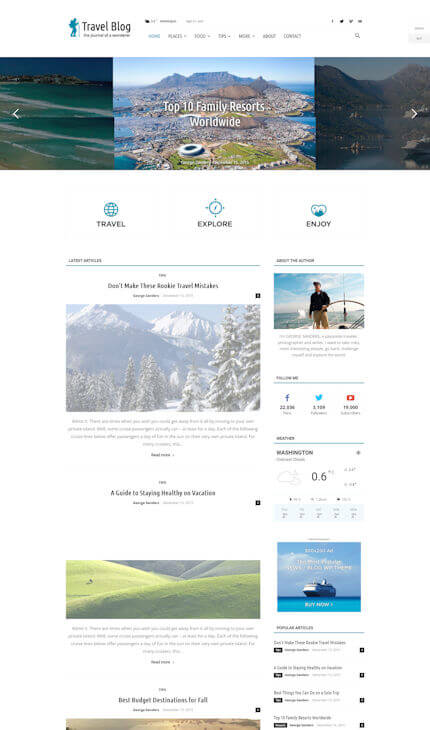This screenshot, taken from the Travel Blog website, features a header with a minimalist icon of a hiker, identifiable by their backpack and walking stick. The top navigation bar includes clickable areas with drop-down menus, as well as icons for various social media platforms.

In the center of the website, a banner highlights stunning imagery. On the left is a serene beach scene, while the far-right showcases a picturesque lake encircled by rolling hills and mountains. Centralized text promotes "Top 10 Family Resorts Worldwide."

Scrolling further down, the site is divided into sections labeled "Travel," "Explore," and "Enjoy," each containing articles, images, and clickable links. One prominent article is titled "Don't Make These Rookie Travel Mistakes," accompanied by a scenic image of a snowy, pine-covered mountainous region. Additional images include a man sailing and various other travel-related visuals and links.